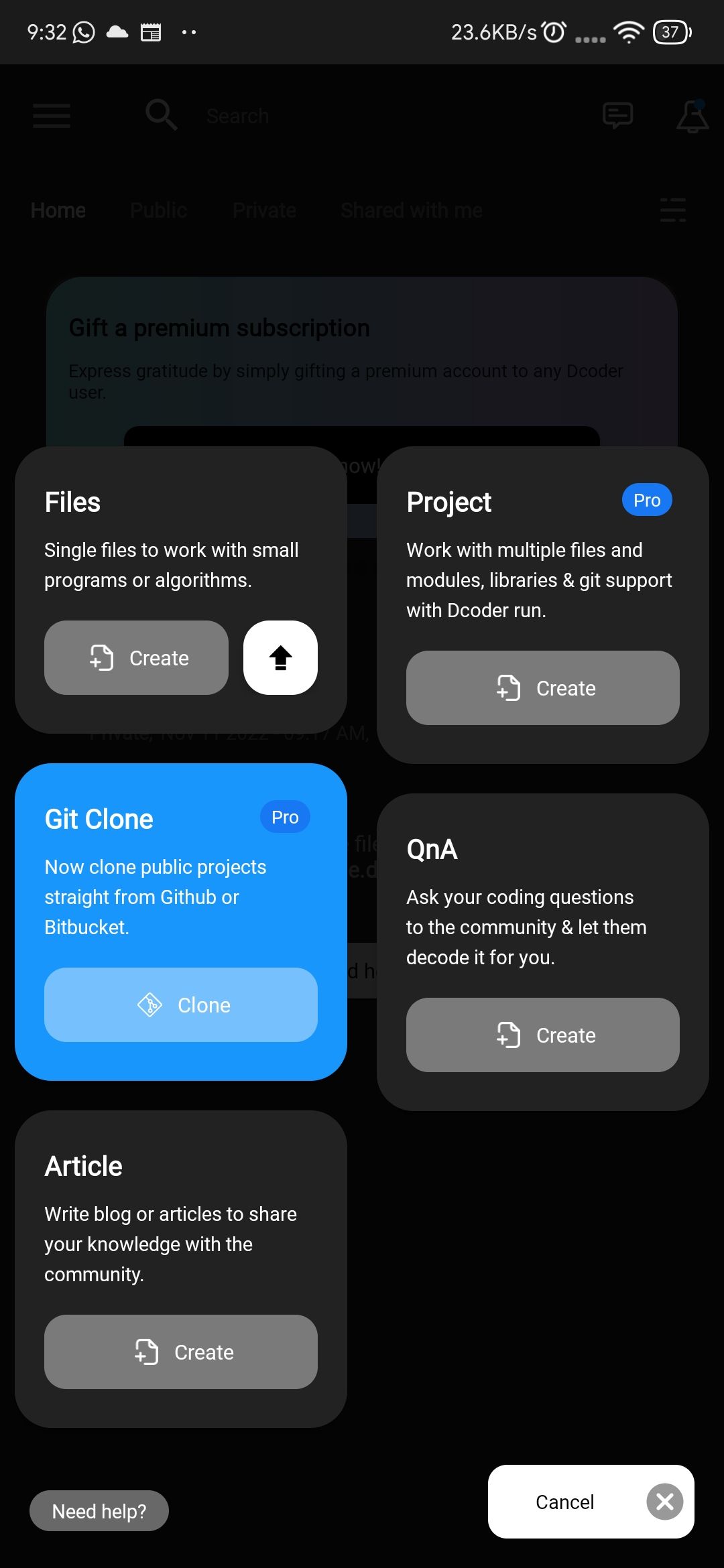A smartphone screen displaying a webpage is captured in this image. The phone's status bar at the top left shows the time as 9:32 AM, a voicemail icon, a battery level of 30%, an active alarm, and full signal bars. The background of the webpage is black. 

In the upper left corner of the screen, there is a dark gray box with white text reading "Files." Below this heading is a description: "Single files to work with small programs or algorithms." Adjacent to this, a light gray button labeled "Create" and a white button featuring a black upward-facing arrow are visible.

Further down, there is a light blue box containing a white text description: "Git clone: now clone public projects straight from GitHub or Bitbucket." This section includes a light blue button with the word "Clone" in white, and a smaller dark blue button with the word "Pro" also in white.

Beneath this section, another dark gray box appears with the white text "Article," accompanied by a description: "Write blogs or articles to share your knowledge with the community." This section includes a light gray button, which is partially cut off in the image.